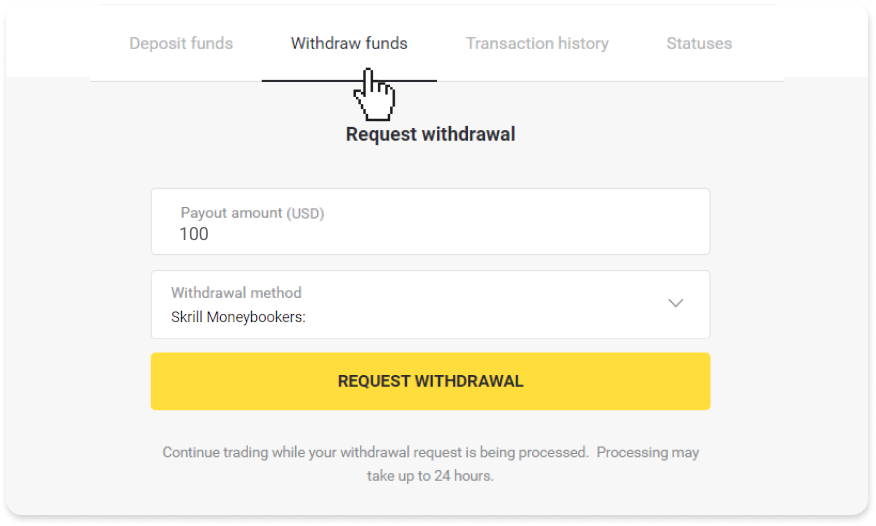In this image, a webpage is displayed with a primary focus on financial transactions. The header of the page includes options such as "Deposit Funds," "Withdraw Funds," and "Transaction History." The cursor is highlighted over the "Withdraw Funds" section, indicating that this is the active page currently in view. Below the header, several details regarding the withdrawal process are listed. These include options for payout amounts, specifically highlighted at USD 100, and the available withdrawal methods, which are "Creel" and "Moneybookers." There is a prominently shown "Request Withdrawal" button, accented in black text on a yellow bar. Towards the bottom of the page, a message is displayed: "Continue trading while your withdrawal request is being processed. Processing may take up to 24 hours." The overall page design features a white background with a black and yellow color scheme, creating a clear and visually appealing interface.